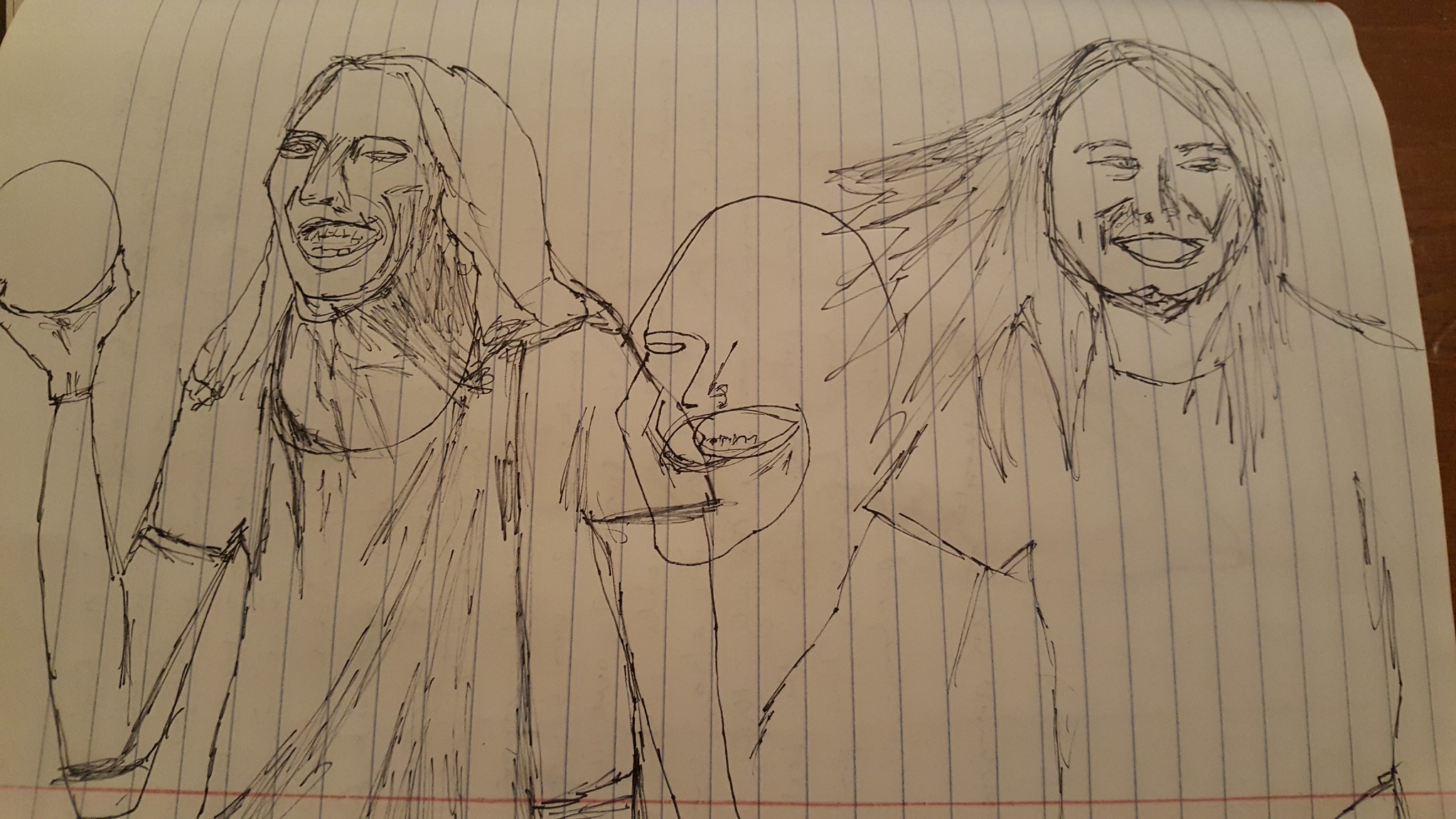The image depicts three distinct ink sketches of a woman on lined notebook paper, bound in a binder. 

- On the left, the woman, wearing a low round-neck short sleeve top, is shown holding a small spherical object in her right hand, palm up, with a soft smile on her face.
- In the center, an initial attempt at drawing her face is evident.
- To the right, the same woman is portrayed with her face slightly turned to the right, wearing a crew-neck short sleeve top, her hair flowing to the left, and a broad smile enhancing her features.

The sketches are arranged horizontally, showcasing different stages and angles of the subject.